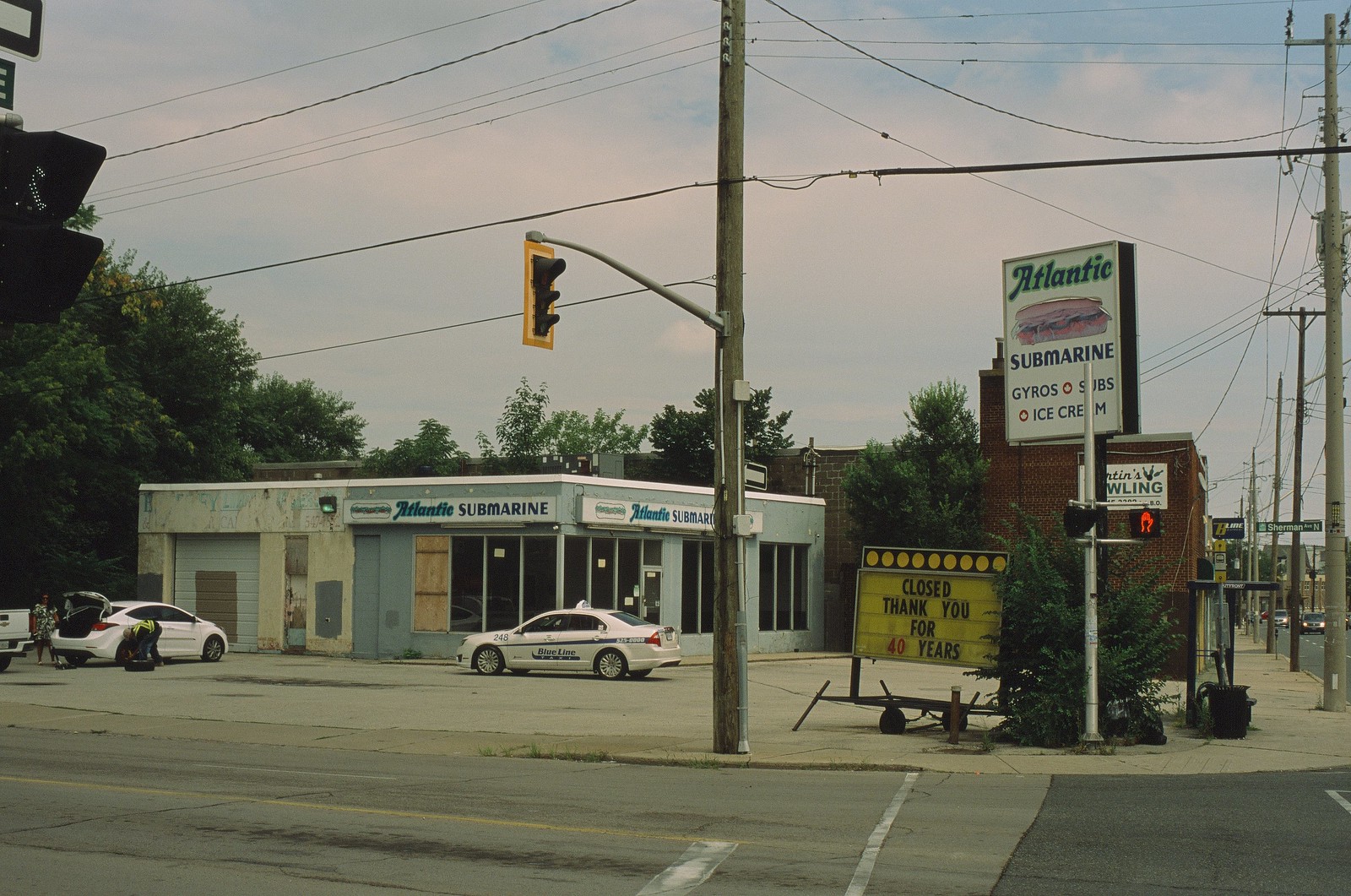The photo captures a somewhat rundown intersection in a small town, focusing on a small corner building housing a sandwich store called "Atlantic Submarine." This store, marked by signs with peeling paint and boarded-up windows, prominently displays its name on both sides of the building. A notable billboard near the street also advertises "Atlantic Submarine," featuring images of gyros, subs, and ice cream. Below this billboard, a yellow neon sign declares the store closed, thanking patrons for 40 years of service. In front of the store, a blue line security vehicle is parked, with additional cars and a taxi with the number 248 parked nearby. In the background, utility poles with wires crisscross above, and traffic lights stand at the intersection labeled as Sherman Street. The scene also features some additional buildings, a few trees, and a lady standing outside a white sedan while another person fixes its tire.